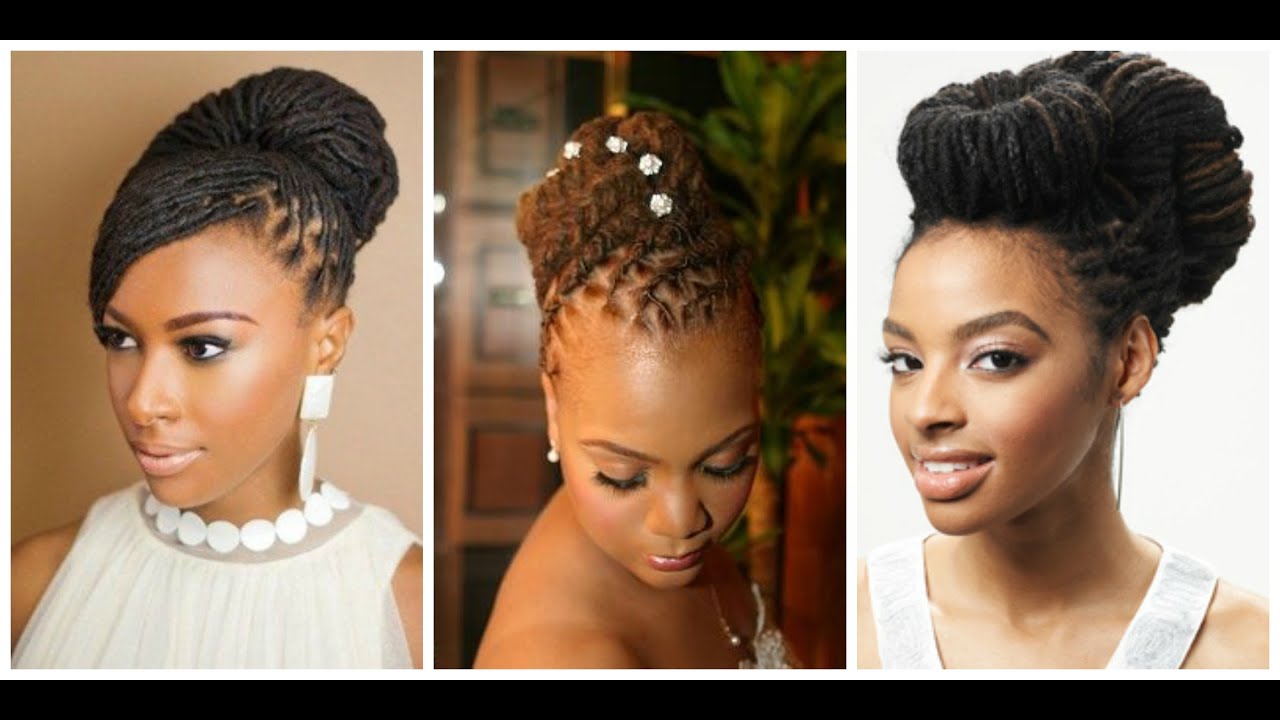This advertisement features three African American female models, each showcased in separate panels with distinct up-do hairstyle designs, emphasizing their individual looks. All three women have caramel-colored skin and dark braided hair, with varying degrees of highlights and accessories. Framed by black bars at the top and bottom, the image brings focus to the intricate details of each model's style.

In the left panel, the first model is looking to the side, revealing her cheek and smile. She has brown extensions woven into a bun and sports long white earrings, a prominent pearl necklace, and a white strapless dress.

The middle panel highlights a model with her eyes closed, gazing downwards. Her light brown braided hair includes beads and is styled neatly, matching her white pearl earring that peeks through as she tilts her head.

On the right, the third model faces the camera with a gentle smile. Her hair is fashioned into two tight buns—one atop her head and one at the back—complementing her caramel skin tone and white tank top.

This image effectively showcases the versatility and elegance of braided up-dos, making each style distinct yet cohesive.